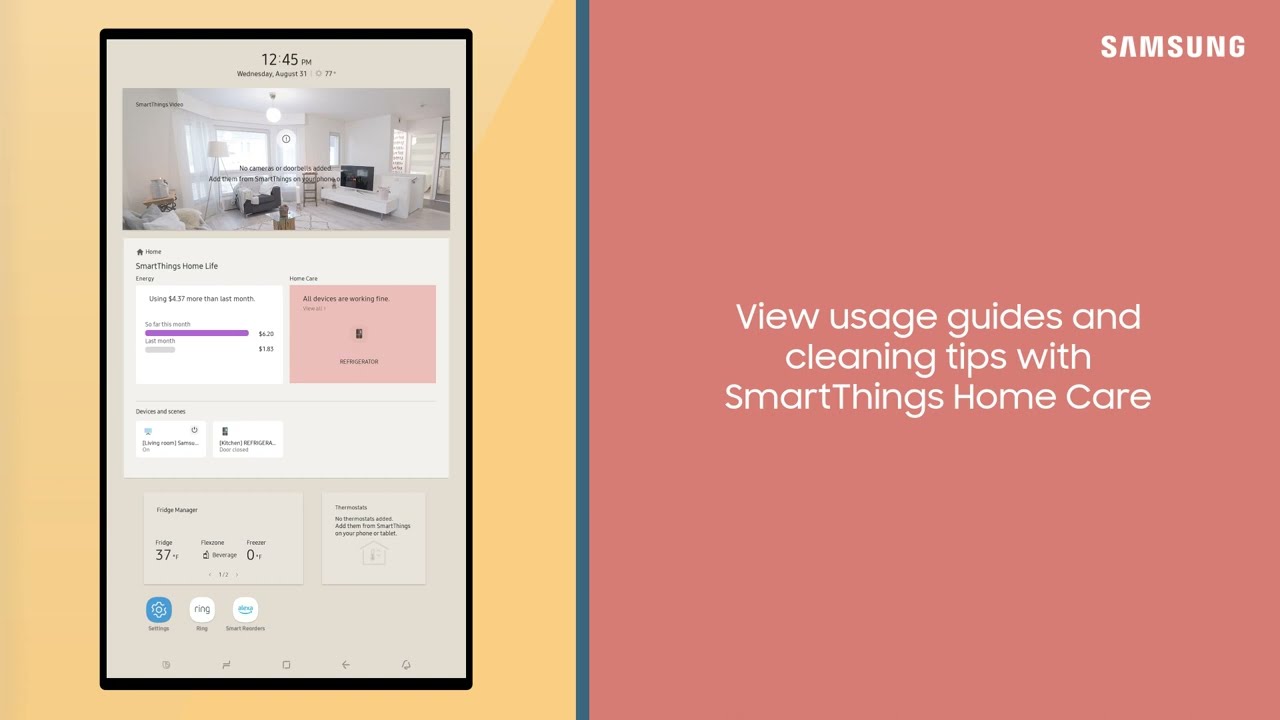The image depicts a Samsung promotional poster divided by a bold blue line into two sections, with the right side larger than the left. The left side features a yellowish-orange backdrop with a black-bordered rectangular frame at the top displaying the time "12:45 PM" and an image of a white living room with white furniture and minimal dark accents. Beneath the picture, the text reads "SmartThings Home Life," followed by two white rectangular boxes containing additional information and two smaller white rectangular boxes below them. At the bottom, there are three circle-shaped icons—one blue and two white. 

The right side of the poster features a pinkish frame with the Samsung logo in bold white letters at the top right corner. Below, the title "View Usage Guides and Cleaning Tips with SmartThings Home Care" is written in white text, emphasizing the promotional nature of the SmartThings Home Care products. This part of the poster is likely representative of an informational or cover page related to Samsung's SmartThings Home Care line. The overall design suggests this is a screenshot or graphic from a Samsung product instruction booklet or app screen.